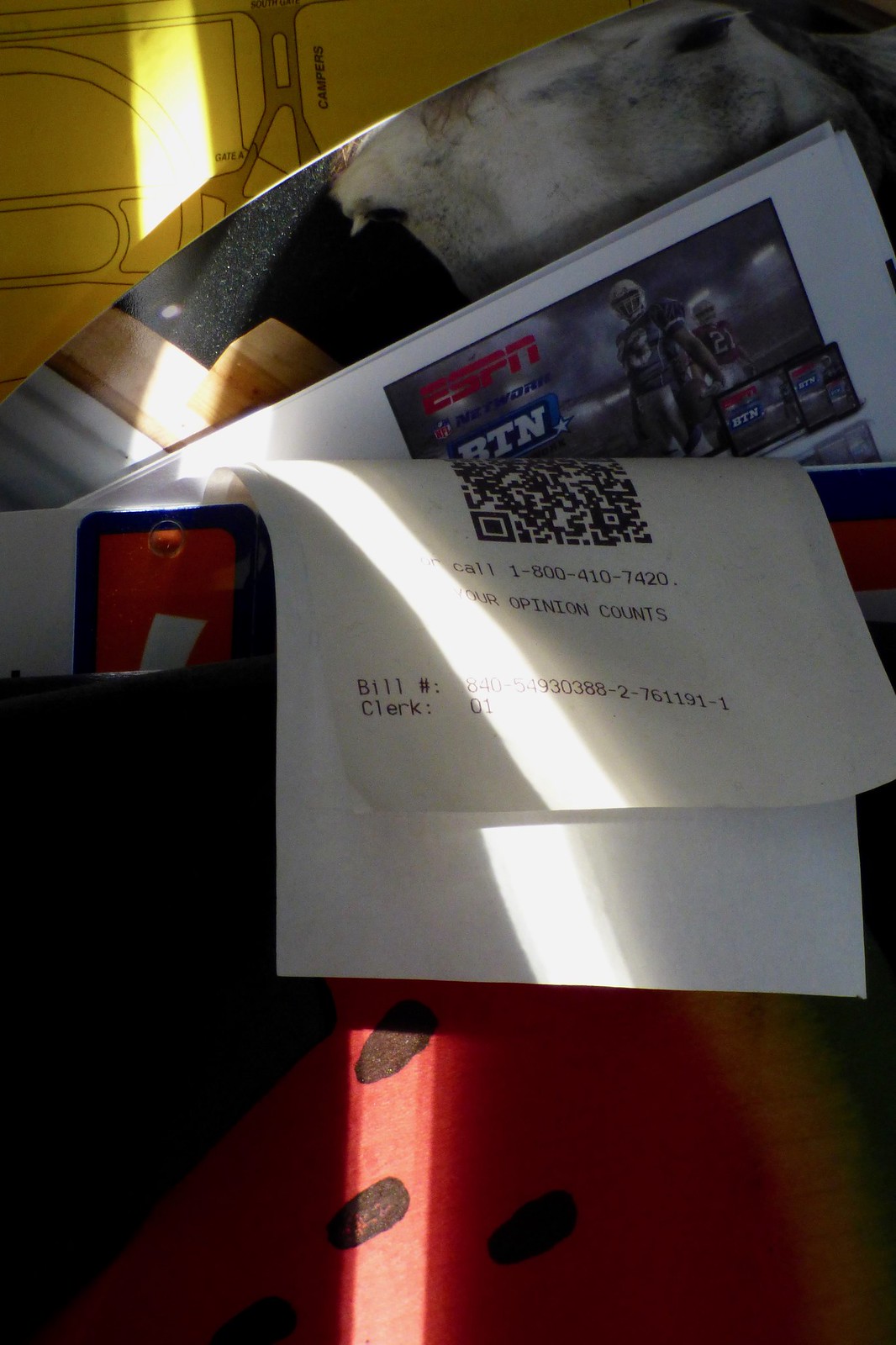This indoor photo captures a small storage pocket overflowing with various papers and documents, some of which are peeking out from the top and are folded over. The topmost paper prominently features a barcode and a number, reading "1-800-410-7420." Additionally, there is an "Opinion Counts" bill marked with the number "840-549-3088-2-761191-1" and a clerk ID labeled as "1." Behind this assortment, a stack of magazines is visible within the diminutive compartment. Also discernible in the backdrop is a poster, with a glimpse of a yellow map perched at the top. The pocket itself is distinctively designed with a pattern reminiscent of a watermelon, characterized by its red color dotted with black seed-like spots.